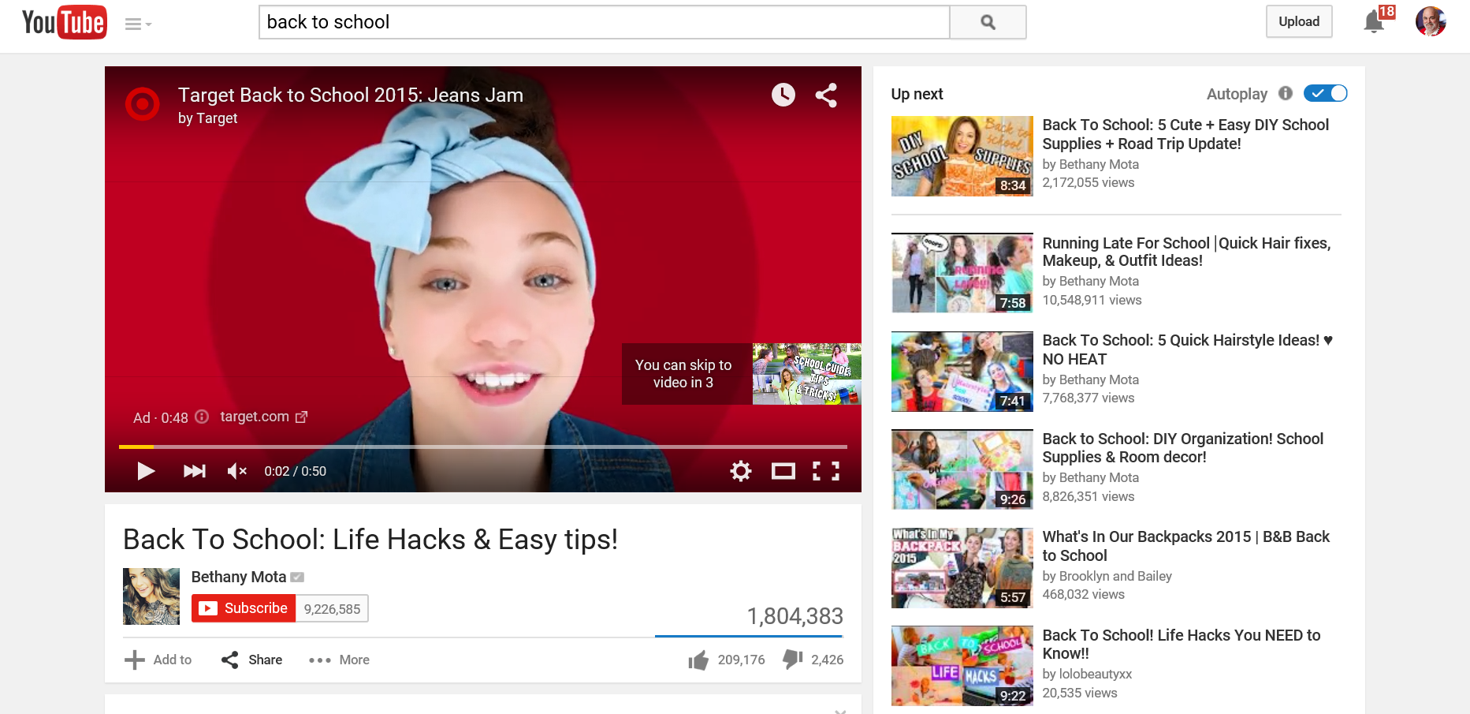This is a screenshot of the YouTube website featuring an advertisement by Target titled "Target Back to School 2015 Jeans Jam." The ad, which is 50 seconds long, is currently 2 seconds in and captures the face of a young girl who appears to be about 15 or 16 years old. She is adorned with a large bow tied as a headband, with her hair styled up, and she is wearing a denim shirt. Her striking light blue eyes are a focal point of the image. The familiar Target bullseye logo is visible in the background. The YouTube interface indicates that the ad can be skipped in 3 seconds, suggesting the viewer was trying to watch a different video titled "Back to School Life Hacks and Easy Tips" by Bethany Mota. The video shows a high number of views, many thumbs up, and some dislikes. On the right-hand side of the screenshot, there are suggested videos, all related to back-to-school outfits and similar topics. The subscribe button for Bethany Mota's channel is also visible.